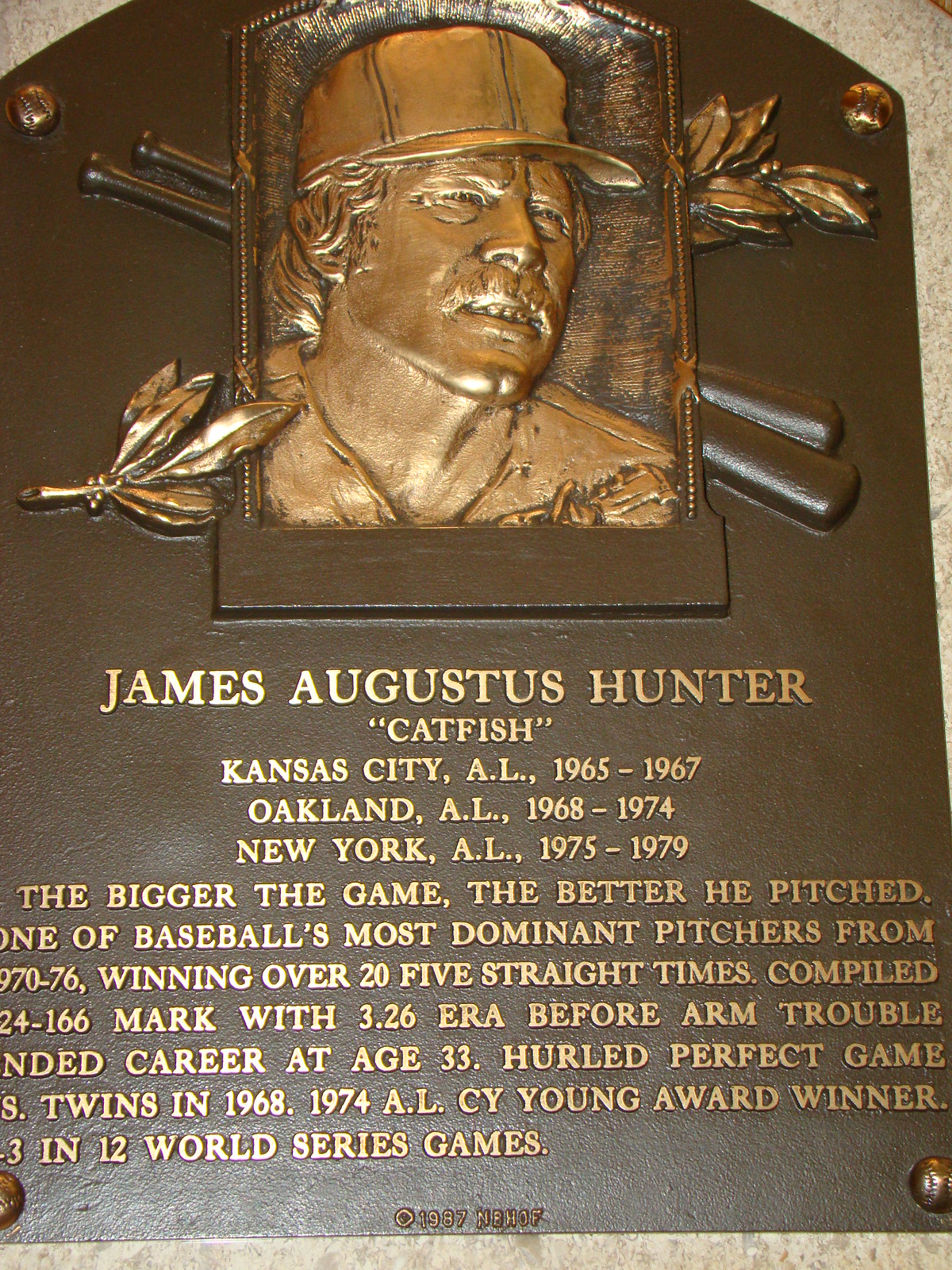The image is a portrait-oriented, color photograph showcasing a bronze memorial plaque, likely located at the Major League Baseball Hall of Fame. The arched top plaque prominently features a raised bronze relief of James Augustus Hunter, known by the nickname "Catfish." Hunter is depicted looking up and to the right, wearing a baseball cap and uniform, complete with a mustache and long hair. Behind his image are two crossed baseball bats and a gold leaf stem. His name, "James Augustus Hunter," is inscribed below the portrait in raised golden lettering. The plaque details his impressive career, listing the teams he played for: Kansas City (AL) from 1965-1967, Oakland (AL) from 1968-1974, and New York (AL) from 1975-1979. Additional text highlights his achievements, such as being one of baseball's most dominant pitchers from 1970-76, winning over 20 straight games, and compiling a notable 224-166 record with a 3.26 ERA before his career was cut short by arm trouble at age 33. Among his accolades, he hurled a perfect game and won the 1974 AL Cy Young Award. The plaque is mounted on a beige marble surface and is designed in a style that combines photographic realism with representational elements.